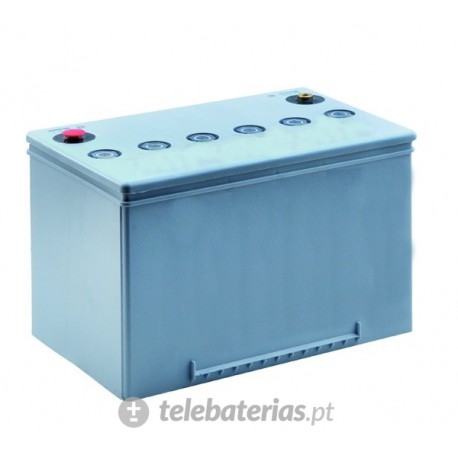The image depicts a light blue rectangular electronic device, likely a battery unit, positioned against a solid white background, giving it a floating appearance. The box is taller and longer than it is wide and is oriented facing southeast. The device, which appears to be made of plastic, features a lid on the top. Centrally aligned on the lid are six light blue circular buttons arranged horizontally. In the top left corner of the lid, there's a red button bordered by a black circle, and in the top right corner, there is a silver knob, also surrounded by a black circle. At the bottom front of the box, there is a grate. Below the box, there is a semi-transparent gray watermark that reads "telebaterias.pt". Accompanying this text is a gray circular logo featuring a white plus sign above a white minus sign.